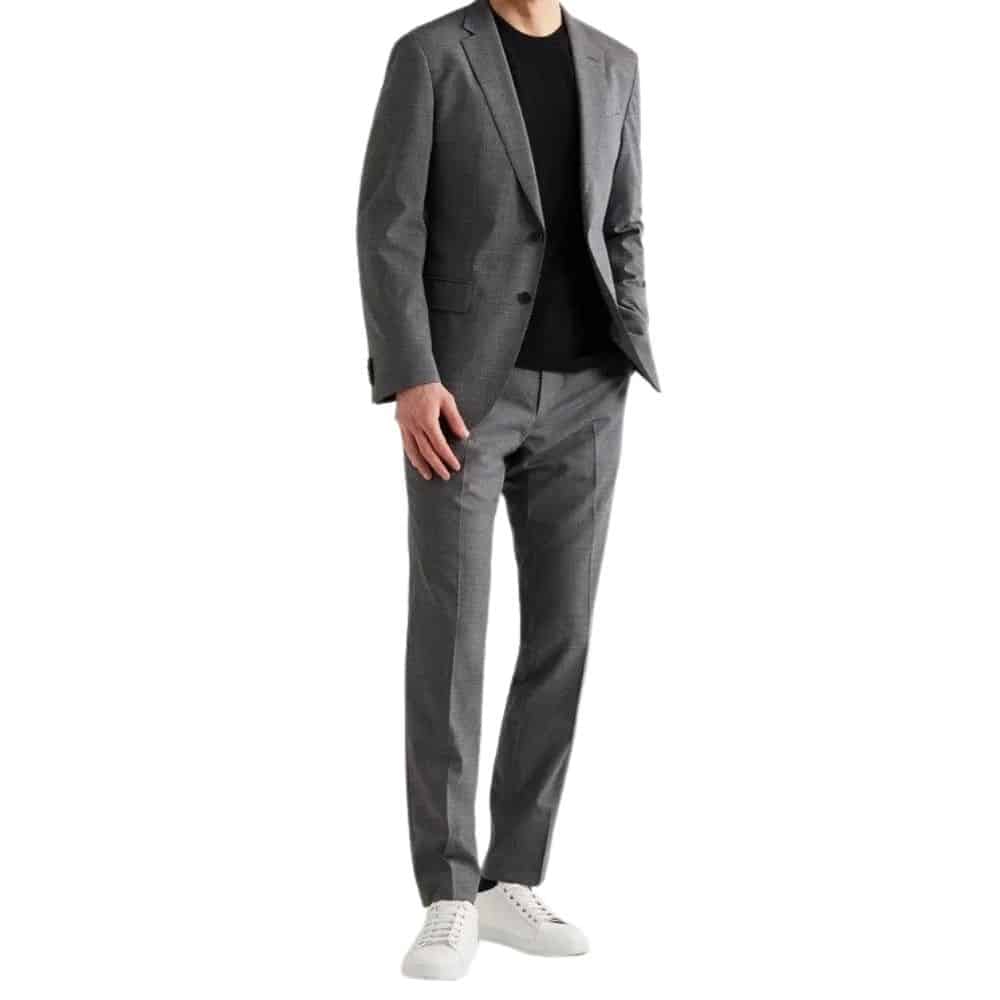The image is a vertically rectangular, professional photograph showcasing a Caucasian male model, cropped from the neck down, with no borders or text around the image. The man is dressed in a dark gray, two-button suit jacket paired with matching pleated slacks. Underneath the suit jacket, he wears a black crew-neck t-shirt, adding to the business-casual aesthetic. His left hand rests casually in his pocket while his right hand is placed on his thigh, slightly exposed along with the skin on his neck. Completing his outfit are white tennis shoes with matching white laces and soles, providing a comfortable yet stylish contrast to his polished attire. The focus of the image is clearly to highlight the high-quality clothing in a meticulously posed manner, suitable for a fashion showcase.